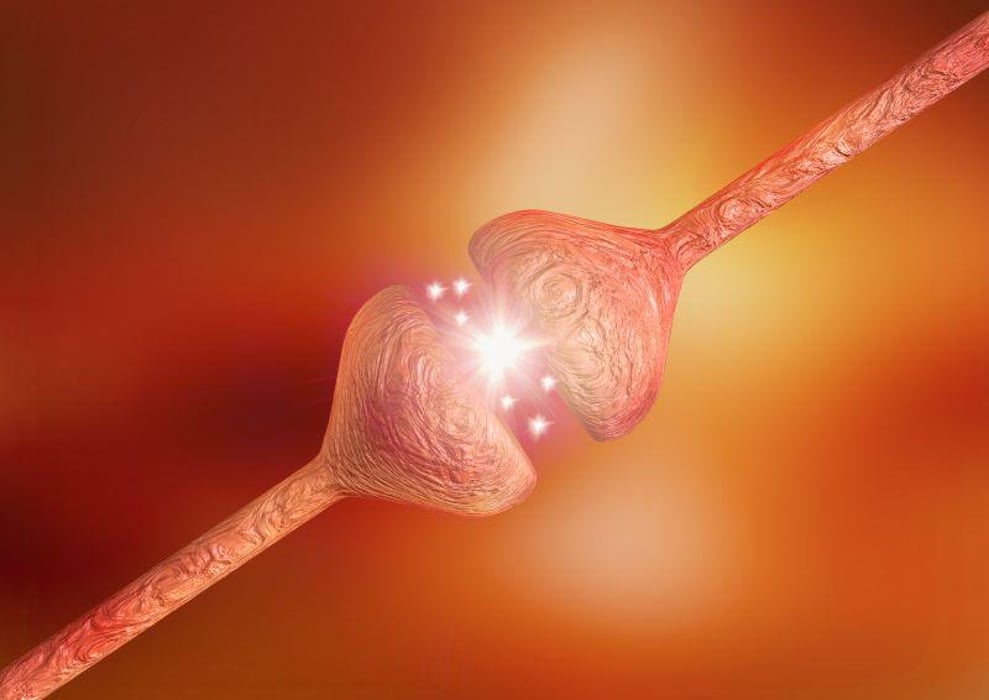The image depicts two neuron-like objects set against a richly toned, orange background. These neuron structures, resembling Hershey Kisses with long, bumpy stems, are positioned diagonally from the lower left to the upper right, nearly touching but separated by a slight gap. The neurons appear to be made of a textured, brain-matter-like material, with an orange-pink, wrinkly surface. At their tips, bright white sparks and stars illuminate the small space between them, suggesting an active electrical connection or neural firing. The background shifts from darker orange and black tones to lighter yellows near the center, emphasizing the luminous interaction between the two neuron-like forms.